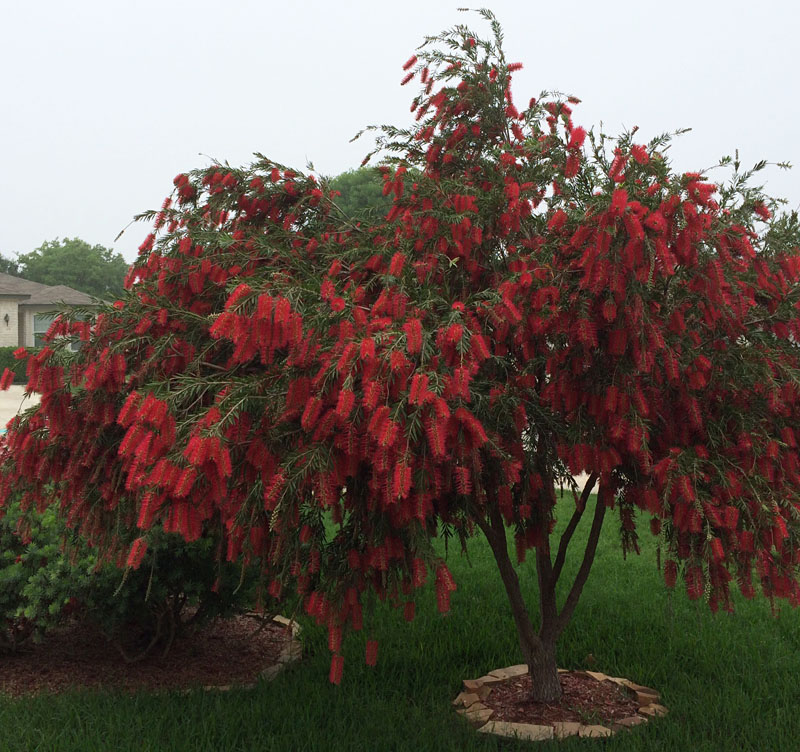This photograph showcases a striking bottle brush tree prominently displayed in a well-maintained yard. The tree is medium-sized, more substantial than a bush, with a prolific, full canopy that extends both high and wide. Its branches are adorned with vibrant red, brush-like flowers, resembling decorative ornaments, hanging gracefully similar to the tendrils of a weeping willow. The vivid red hues contrast beautifully with the lush green foliage, evoking festive Christmas colors. The area around the tree is carefully landscaped with a rock border and mulched base, emphasizing its manicured setting. The yard itself features rich green grass and additional green shrubs similarly landscaped with stone and bark. In the background, one can glimpse a house and walkways, confirming the residential nature of the scene, while a house and what appears to be a driveway are subtly visible through the trees.